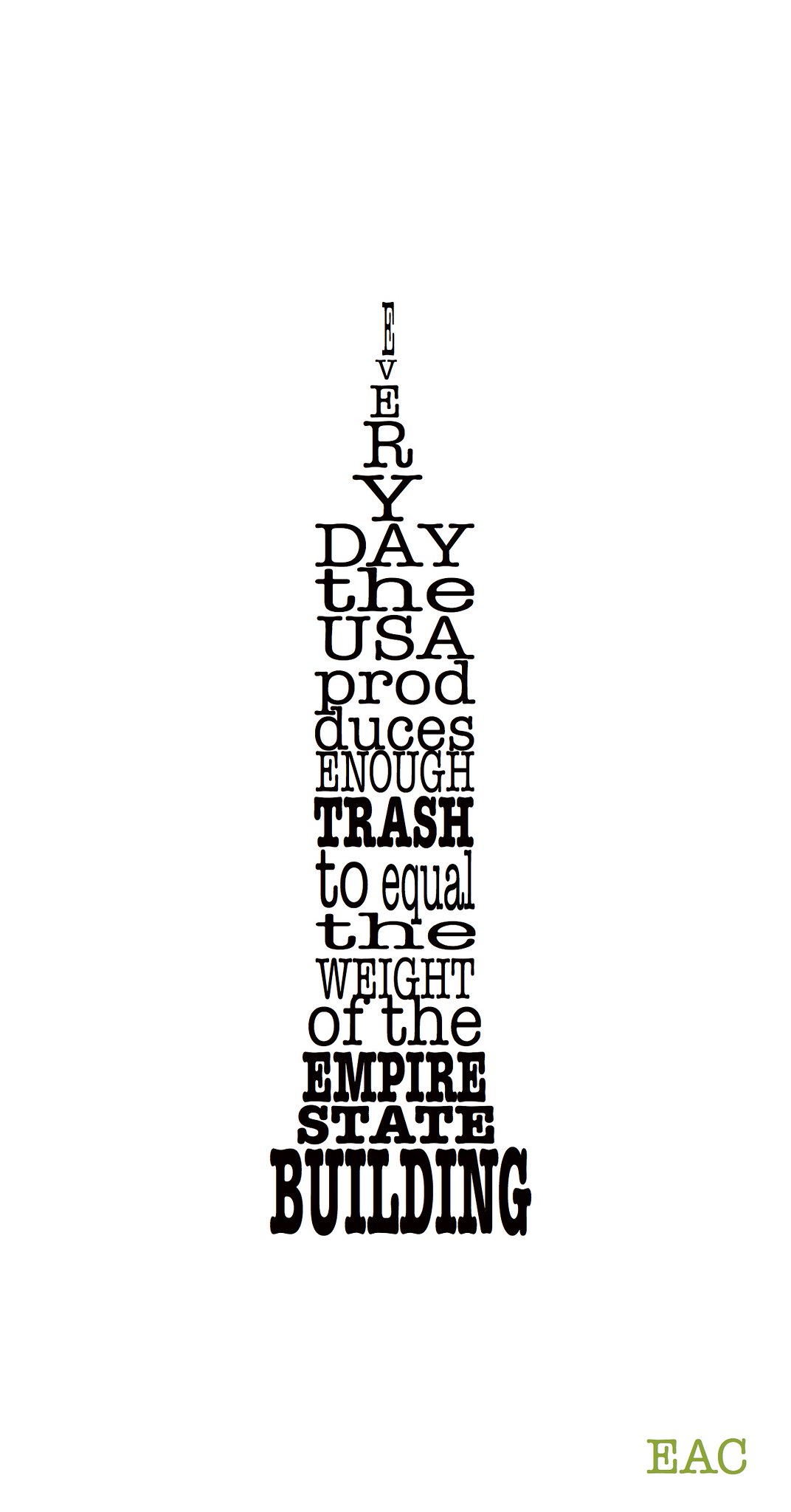This image depicts the iconic shape of the Empire State Building, but instead of being a traditional photograph, the structure is cleverly composed entirely of black text. The text itself conveys a stark message: "Every day, the USA produces enough trash to equal the weight of the Empire State Building." The words are arranged vertically, starting from the pinnacle with the letter "E" and progressively getting larger as they descend, mimicking the form of the tower, which is rectangular at the base, slightly narrowing before finishing with a spire at the top. The font used throughout is black and appears to resemble a typewriter style, such as Times New Roman with varying thicknesses for emphasis. The entire composition sits against a completely white background, emphasizing the text-formed tower. Additionally, in the bottom right corner, the letters "EAC" are prominently displayed in green, possibly serving as a watermark or signature.